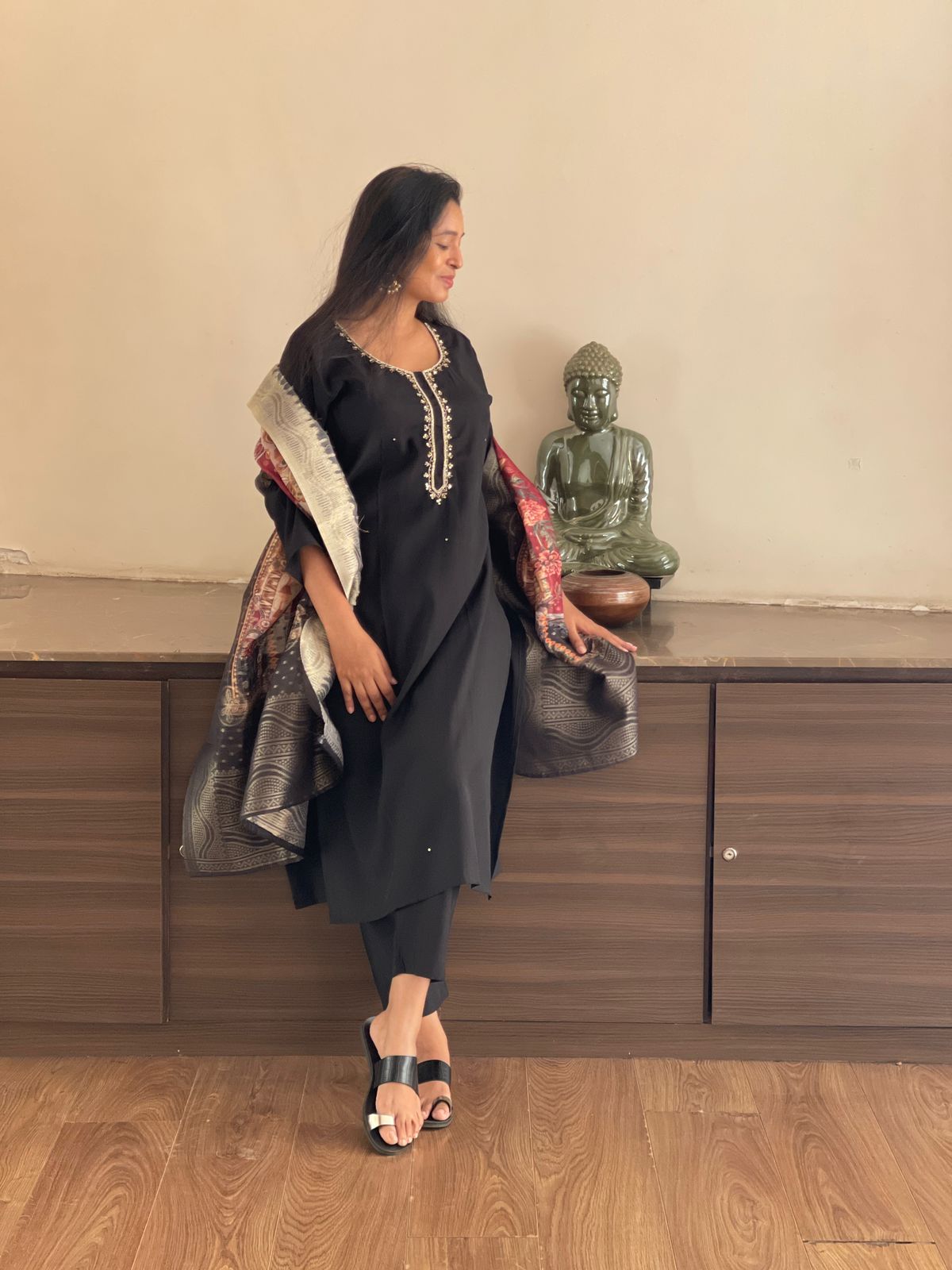The photograph features an Indian woman standing on a wooden floor, which occupies the bottom third of the image. She is leaning against a long, low wooden cabinet with her hands resting: one on her lap and the other gently touching the back of the cabinet. The cabinet, or chest drawer, is topped with a small opal Buddha statue in the lotus position and an ashtray in front of it. The woman is dressed in traditional Indian attire: a black top with a mid collar, black pants, and black sandals with a distinctive white strap around the left toe and a black strap around the right toe. She is also wearing a multi-colored cover-up with gold trim and accents of orange and red, which is draped behind her shoulders but rests over her elbows. Her long hair frames her face as she gazes to her left, displaying a calm profile. She completes her look with long earrings. The background includes a white wall behind the dark wood-colored cabinet, adding contrast to the scene.